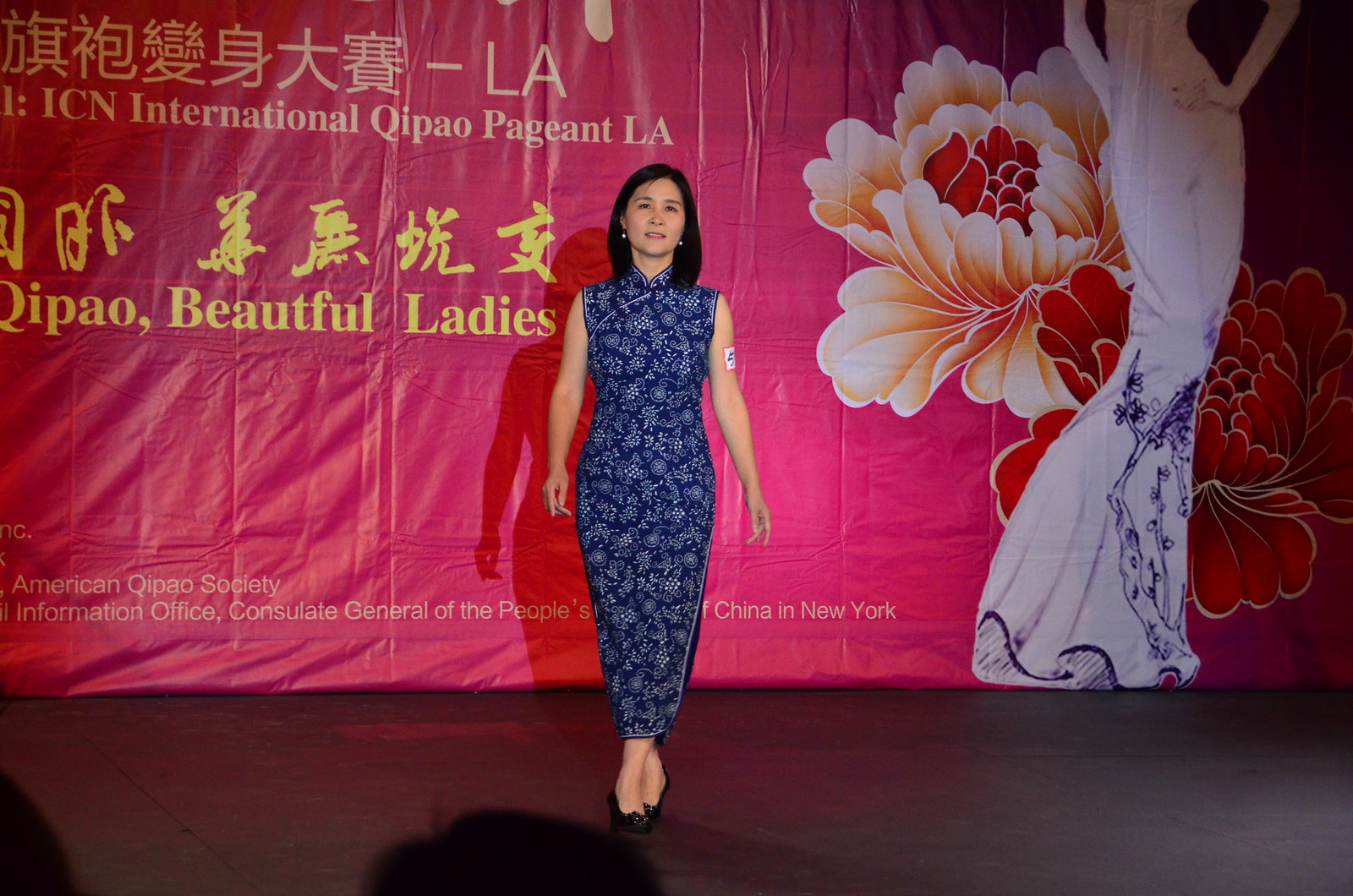In this image, a woman stands center stage, wearing a form-fitting blue dress styled like a kimono. Behind her, a vibrant red poster adorned with floral motifs and a tree—or possibly another woman—is prominently displayed. The poster reads "ICN International Qipao Pageant LA" followed by Chinese characters, and additional text stating "Qipao Beautiful Ladies" and "American Qipao Society, Information Office, Consulate General of the People's Republic of China in New York." The stage setup includes a curtain in the background, and glimpses of a hard or lightly carpeted floor. At the bottom of the image, the backs of spectators' heads are visible. The scene is well-lit, suggesting the event is indoors, though details about the time of day are unclear. The woman on stage, who appears to be part of a judging segment, looks elegant and wears a sticker on her arm. The backdrop and attire are highlighted by an array of colors including black, gray, blue, light blue, pink, yellow, red, orange, and purple.